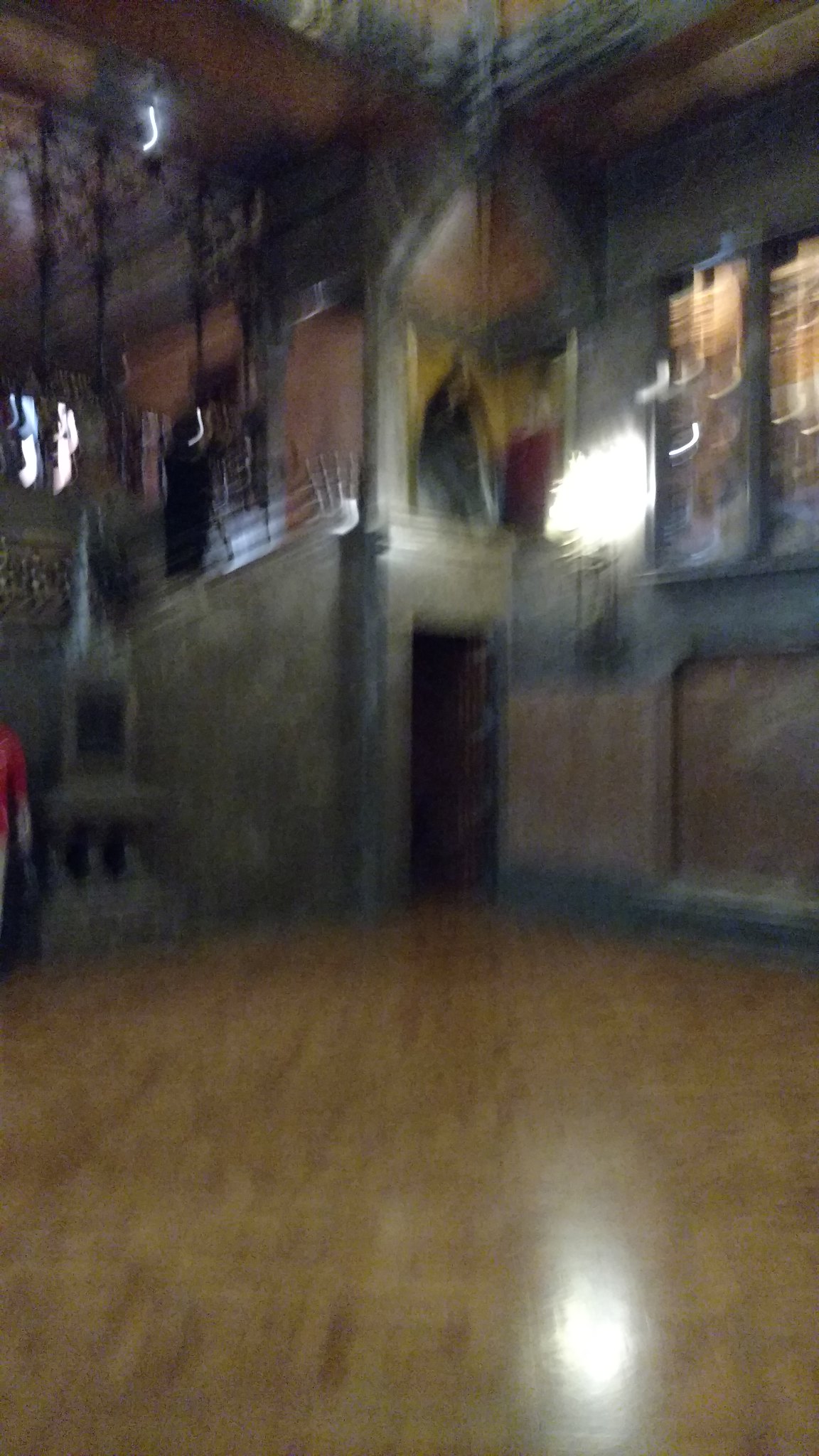The image captures a dimly-lit interior of a religious building, likely a chapel or an old church. On the right-hand side, a biblical painting is mounted on the wall, depicting two figures kneeling—one in red attire and the other draped in a grey shawl. Beneath the painting, a robust wooden door is noticeable, leading to a polished wooden floor. In the mid-left section, a small stone structure resembling a temple stands, adorned with elaborate decorations hanging from the ceiling above. The overall dark ambiance adds to the solemn and sacred atmosphere of the scene.